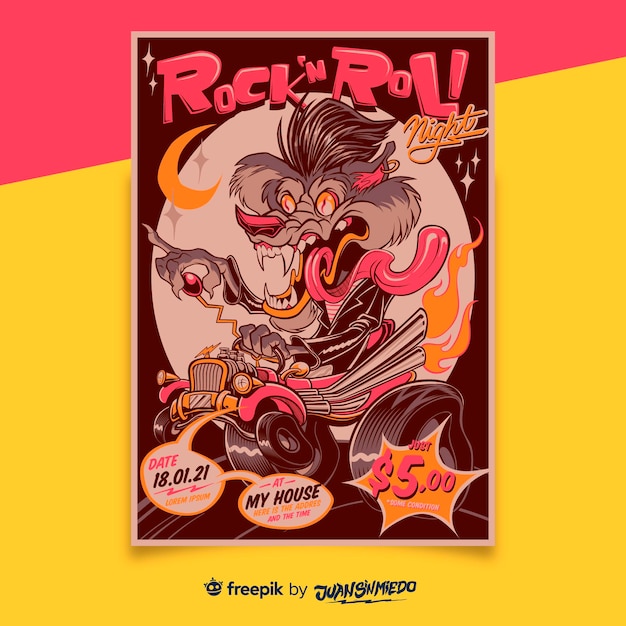The image is a vibrant rock-and-roll concert poster set against a striking background divided diagonally, with the top tenth in bright pink and the bottom in mustard yellow. A dynamic cartoon wolf with exaggerated features, pink nose, ears, and a swirling tongue, drives a hot pink muscle car with silver exhaust pipes spewing fire. The wolf wears a black leather jacket over a pink and white striped shirt, and grips the gear shift with its pinky raised. The car’s headlights resemble eyes, adding a whimsical touch. A full moon looms behind the wolf, enhancing the night-time setting. At the top of the poster, “Rock and Roll” is emblazoned in hot pink with an exclamation point, and below it, “Night” is written in cursive yellow. Other details include a burst of pink text on a yellow background stating, "Just $5," and at the bottom, it mentions "Free Pick by Juan Sin Miedo." Additionally, there are word bubbles around the car’s tires announcing the event date as January 18th, 2021, at an unspecified location, implying, "at my house."